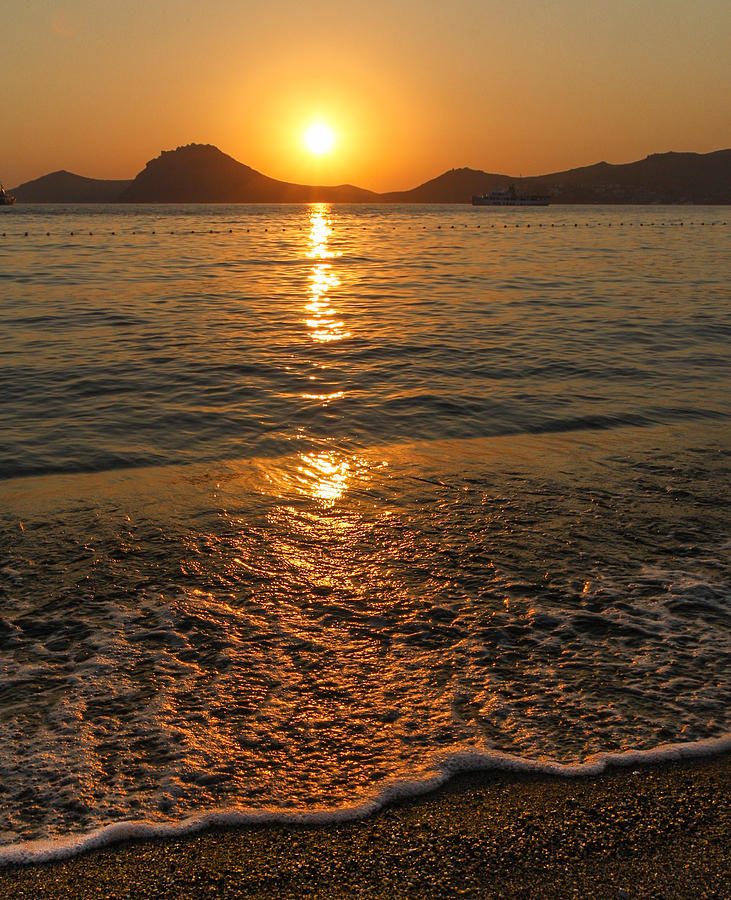The image is a professionally taken, full-color photograph of a serene beach at sunset. The photo, vertically rectangular with no distinctive border, captures a sandy shoreline in the lower section where foamy waves softly kiss the sand. The sand itself is a medley of multiple shades—brown, black, white, gray, and tan—with scattered pebbles adding texture. Moving further back, the calm, metallic gray-blue water stretches to the horizon, where it meets a silhouette of black, hilly landmasses. The sky above the horizon is a mesmerizing gradient of grayish-orange. Just left of the center, the glowing orb of the sun shines brilliantly, casting an orange and yellow halo while reflecting a vivid path of light onto the water. The overall scene is bathed in an orange glow, enhancing the tranquil and picturesque quality of the landscape. The image has no people, animals, or text, and the composition and lighting underscore its professional quality.